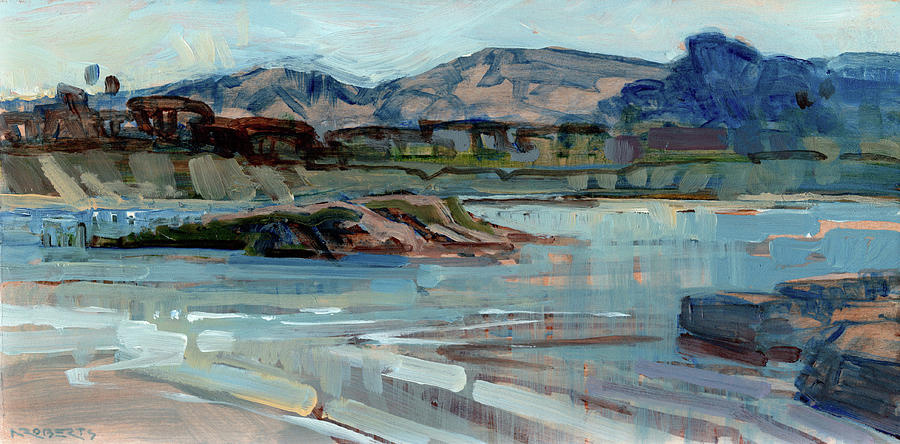The painting, an impressionistic landscape signed by A. Roberts, features a serene scene dominated by a large body of water with an island at its center. The island, predominantly colored in brown and green, rises from a pond or lake that extends across the canvas in varying shades of blue with accents of white. At the water's edge in the background, there is a village or cluster of square, brown structures, representing houses or other buildings. Behind this village, a range of tall mountains stretches across the scene. These mountains show an array of colors, from tans and browns to dark blues. On the right-hand side, a larger, entirely dark blue mountain stands prominently in the foreground, slightly ahead of the others. The sky overhead is a light blue, almost devoid of clouds, enhancing the tranquil atmosphere of the scene. Further foreground elements include a cliff to the left, some tan and blue rocks at the water's edge on the right, and a grayish-peach sandy area peeking out at the bottom left, adding to the complex and textured composition of the painting.